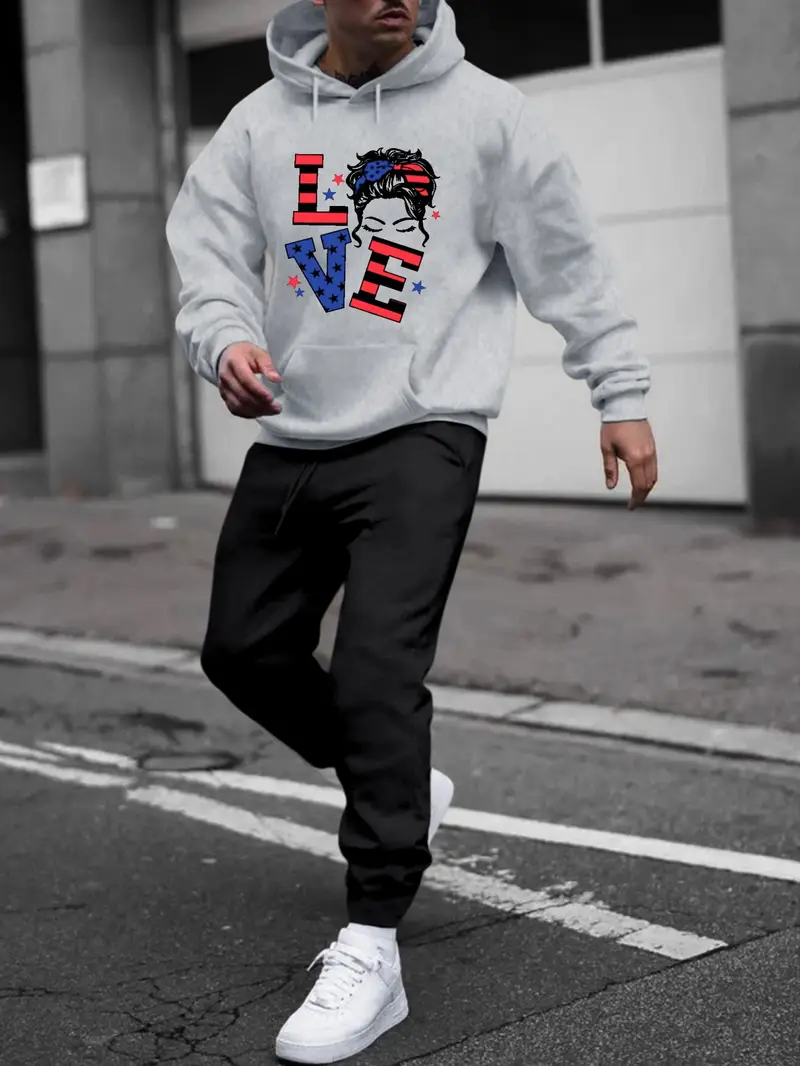In this outdoor daytime photograph, a man, presumably white, is captured mid-stride as he crosses a gray street marked with white lines. His attire includes slightly baggy black sweatpants and white sneakers, with one foot lifted off the ground. He wears a gray long-sleeve hoodie prominently featuring the word "LOVE," where the "O" is creatively replaced with an image of a woman with black hair. The letters "L" and "E" are decorated with orange and black stripes, while the "V" is blue, all contributing to a vibrant and eye-catching design against the hoodie’s gray backdrop. The man’s face is cropped from the nose up, revealing only the lower portion, which includes his mouth and a hint of a mustache. Behind him stands a nondescript gray concrete wall and a pull-up garage door, adding to the image's urban setting.